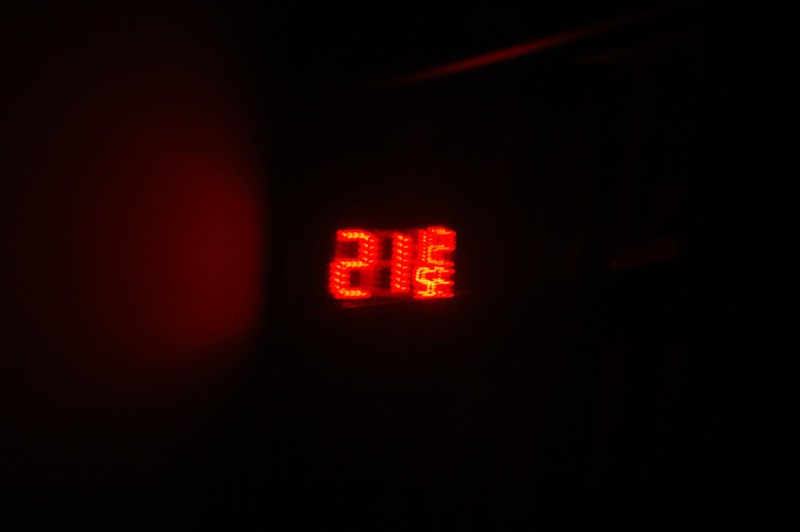In this photograph, we see a dimly lit scene dominated by an extremely blurry image of what appears to be a digital alarm clock, possibly the result of a long exposure. The bulk of this image is pitch black, highlighting the sparse light sources. In the center, a square or rectangular clock displays a series of bright red LED or neon-lit numbers made up of little dots of light. The most discernible digits are a 2 and a 1, with additional numbers stacked below and beside them, possibly reading 12 and 5, though these are quite hard to make out due to the blurriness. The faint reddish glow from the numbers casts subtle light onto the left side of the frame and just a bit in the top right corner, creating a dimly lit silhouette effect on what might be the edges of a wall or ceiling.